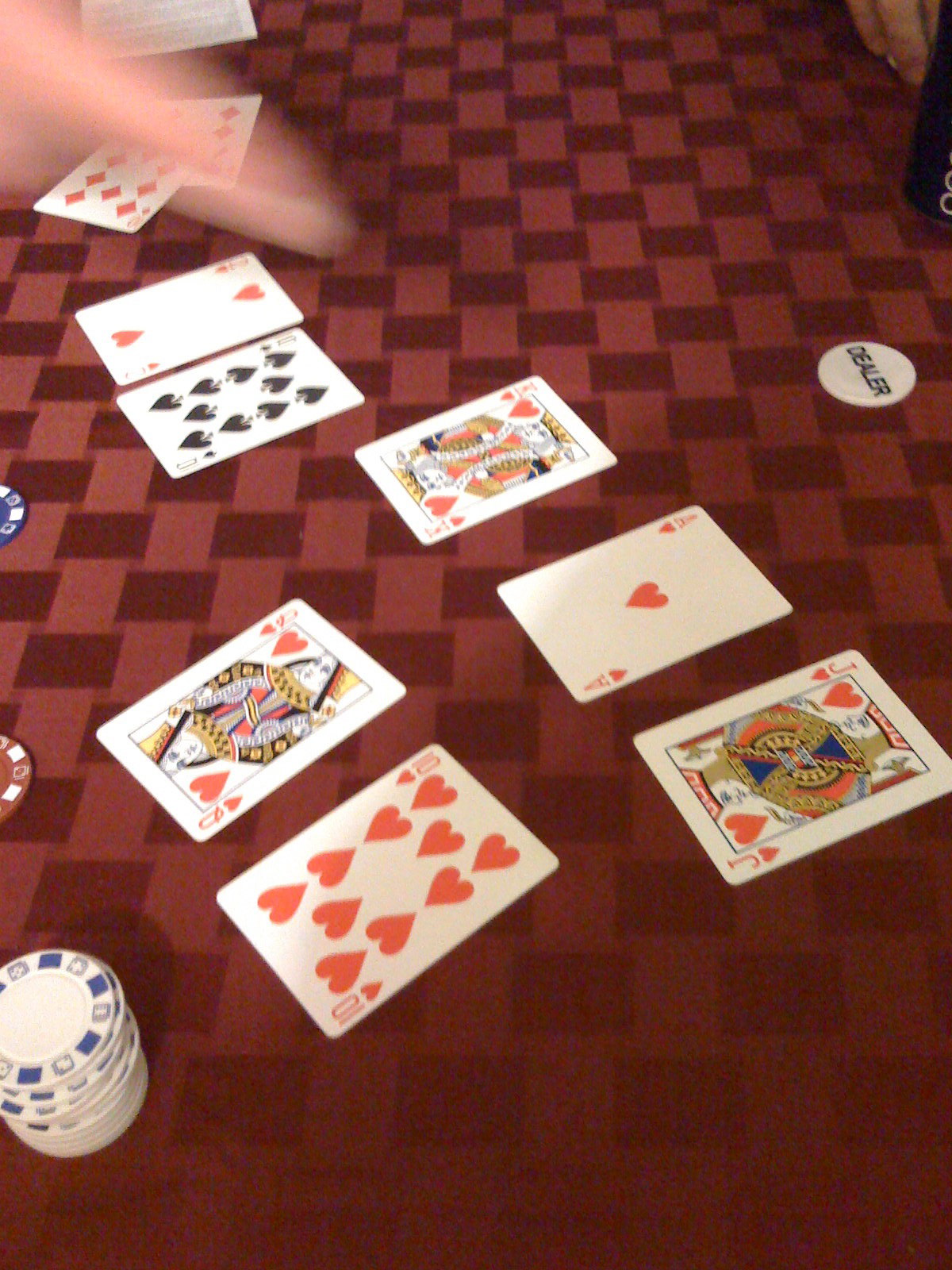In the image, a lively card game is in progress atop a checkered red cloth featuring dark and lighter red squares. Prominently displayed on the cloth are several playing cards: the ten of hearts, the jack of hearts, the ace of hearts, the queen of hearts, the king of hearts, the ten of spades, the two of hearts, and the nine of diamonds. A distinctive dealer chip sits among the cards, highlighting the game's intensity.

To the side, stacks of poker chips are neatly arranged, indicating the high stakes of the game. The chips vary in color and design, featuring white chips with blue markings, a red chip with white markings, and a blue chip with white markings. Adding to the dynamic atmosphere, blurred hands in motion suggest multiple players actively engaged, with one hand clearly visible in the upper right corner. 

In the same corner, a black object partially enters the frame, its identity obscure due to limited visibility. The scene captures the essence of a high-energy gambling experience, replete with strategic plays and betting anticipation.